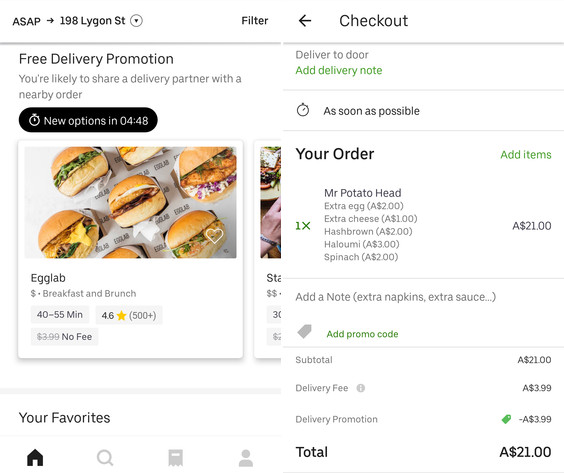The image shows a detailed breakdown of an online food order for delivery from a restaurant named "Egg Lob" located at ASAP198 Leggen Street, which is offering a free delivery promotion and the possibility of sharing a delivery partner with another nearby order. The order interface indicates options for delivery to the door and allows for the addition of delivery notes, requesting the delivery as soon as possible.

The restaurant, Egg Lob, which operates for breakfast and lunch and is identified by a single dollar sign, features prominently on the screen. They specialize in an array of appetizing sandwiches with hamburger buns, which have garnered a high rating of 4.6 stars from over 500 reviews. The estimated delivery time is noted to be between 40 to 55 minutes, and there is no delivery fee due to the current promotion.

The customer has ordered an item named "Mr. Potato Head," customized with extra egg, extra cheese, hash browns, spinach, and what appears to be "el-a-yumi" (a possible typo or local specialty). This customized sandwich is priced at $21. Additional instructions for the order include a request for extra napkins and extra sauce, with a field to input a promotional code.

Summarizing the billing details, the subtotal for the sandwich is $21, the default delivery fee of $3.99 is waived due to the promotion, making the final total $21.